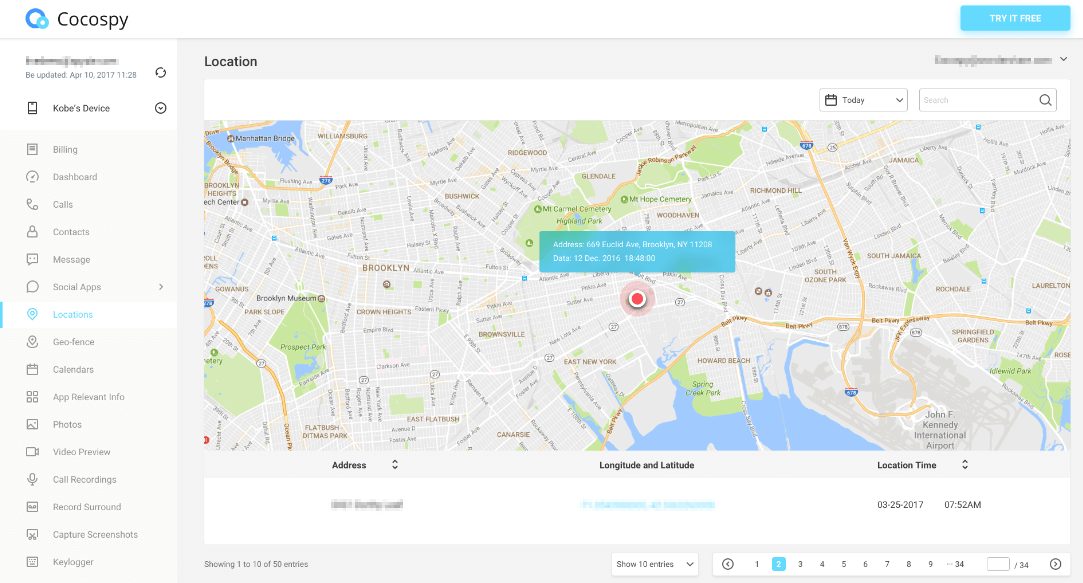On a clean white background, the upper left corner features two overlapping circles: the larger one is a deep blue, and the smaller one, positioned slightly in the bottom right of the larger circle, is a lighter blue. Adjacent to these circles, in bold black text, is the title "Cocoa Spy". The central area of the image is mostly blank with ample white space.

On the right-hand side, there is a prominent blue button with "Try it Free" written in white text. Below, aligned to the left, the white background appears digitally altered, possibly obscuring previous content. Underneath this section, in grey text, it states "re-uploaded" followed by a date. Directly below this, in bold black text, it reads "Kobe's device".

The lower portion of the image features multiple grey text labels arranged in a vertical list over a light grey background. These labels include: "billing", "dashboard", "calls", "contacts", "messages", "social apps", "geofence", "calendars", "app related info", "photos", "video preview", "call recordings", "record sound", "capture screenshots", and "keylogger".

On the far right, a grey background contains a white box with a dropdown menu labeled "Today" beside a search bar. Centrally positioned within this box is a Google Maps-like interface displaying a red marker and overlaid with unreadable blue text.